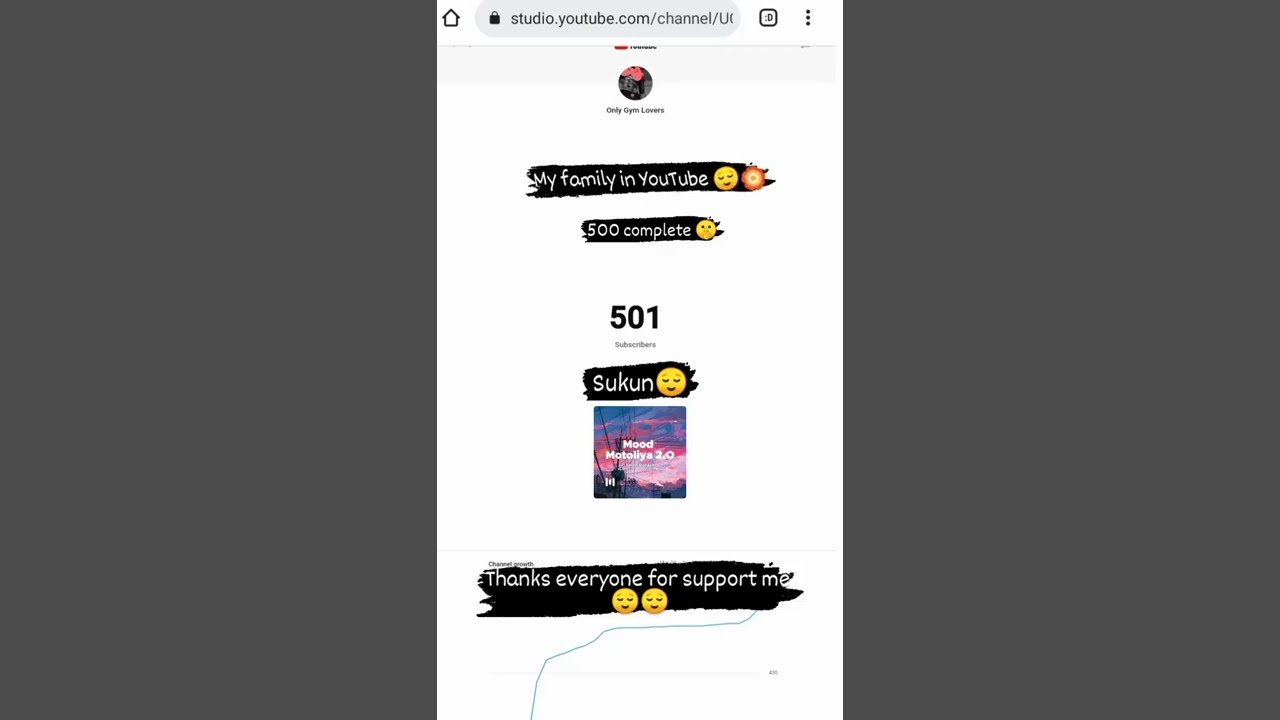This detailed digital image is divided into three panels: the central third showcases a screenshot while the outer two-thirds are dark grey blocks. The screenshot appears to be taken from a smartphone displaying a web page, likely from YouTube Studio. At the very top, a bar is present featuring a home button on the far left, various icons on the far right, and a central grey bar containing a truncated URL: studio.youtube.com/channel/ you... In the top section of the screenshot, part of the YouTube logo is faintly visible, obscured by the bar.

Below this, there's a profile picture depicted as a circle with bright red and dark colors but lacking distinguishable detail. The text "Only Gym Lovers" is printed beneath the profile icon. Further down, the phrase "My family in YouTube" is written in white text on a black background accompanied by a smiley face emoji and a flower emoji. Following this, the text reads "500 complete" alongside a shushing emoji, also in white text on a black background. Underneath, "501 subscribers" is written in black text.

Continuing down, the word "Sukun" with a smiley face emoji appears in white text on a black background. Below it, there is a small square image with the text "Mood Motolia 2.0" set against a sunset with pink and blue hues. The concluding section contains the phrase "thanks everyone for support me" in white text on a black background, followed by two smiley face emojis. A blue diagonal line, ascending from left to right, spans the bottom of the image. The entire screenshot background is flat white.